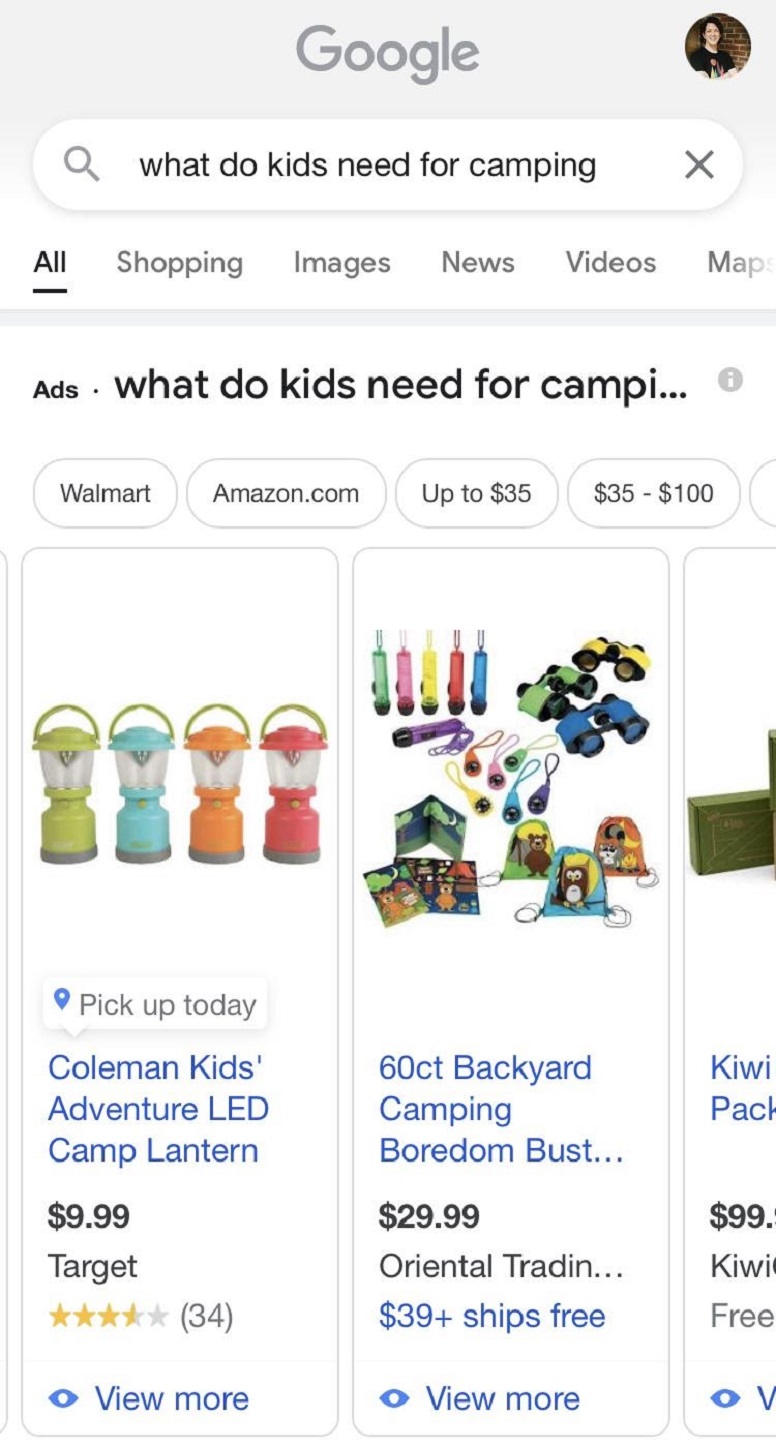This image captures a screenshot of a Google search results page. The header area of the website is light gray, with the Google logo prominently displayed in dark gray text, featuring a capital "G" in the center. 

On the right side of the header, there is a circular user icon. Below the header, a white search bar is visible, containing a gray magnifying glass icon on the left and the search query "what do kids eat for camping" inside. An "X" icon is situated on the right end of the search bar.

Beneath the search bar, a horizontal menu is displayed. The menu options are labeled in bold, underlined text with the first letter capitalized: All, Shopping, Images, News, Videos, and Maps.

The main content area of the page has a white background. The category "Shopping" appears at the top, and the search query "what do kids eat for camping" is shown again along with links to Walmart and Amazon products in varied price ranges. The details are partially cut off.

Further down, there are three product panels, with the third panel partially visible. The first panel displays an image of a Coleman Kids Adventure LED Camp Lantern priced at $9.99 available at Target, along with user ratings from 34 reviewers and a "View More" link. The second panel features a different product: a 60 count Backyard Camping Boredom Bust set priced at $29.99 from Memorial Oriental Trading, noting that orders over $39 ship free and including a "View More" link. 

The third panel is cut off, making its details partially obscured.